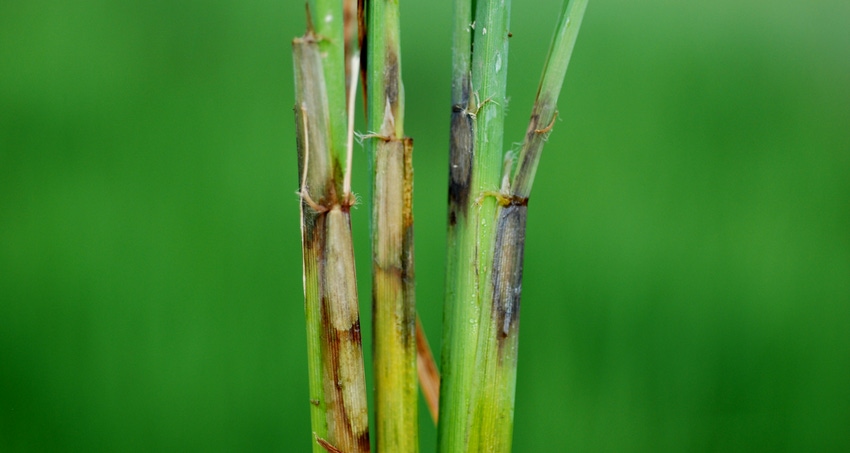This close-up macro photograph features three distinct stalks of a greenish plant, potentially bamboo, emerging vertically and cut off by the frame's top and bottom edges. The backdrop consists of a deep green blur with lighter green splotches in the center and darker hues at the corners, emphasizing the stalks' vivid presence. The leftmost stalk showcases a green stripe and a light brown patch on its lower left, culminating in a very light brown tuft at the top. The middle stalk presents a yellowish-green base with dual black stripes, a light brown triangle midpoint featuring a dark spot above it, and continues in green. The rightmost, thickest stalk is predominantly deep green, marked by a dark gray rectangle near the top left and another in the middle right, suggesting signs of decay or damage, as indicated by numerous lesions and dark spots, enhancing the image's visual narrative of aging or illness within the plant.